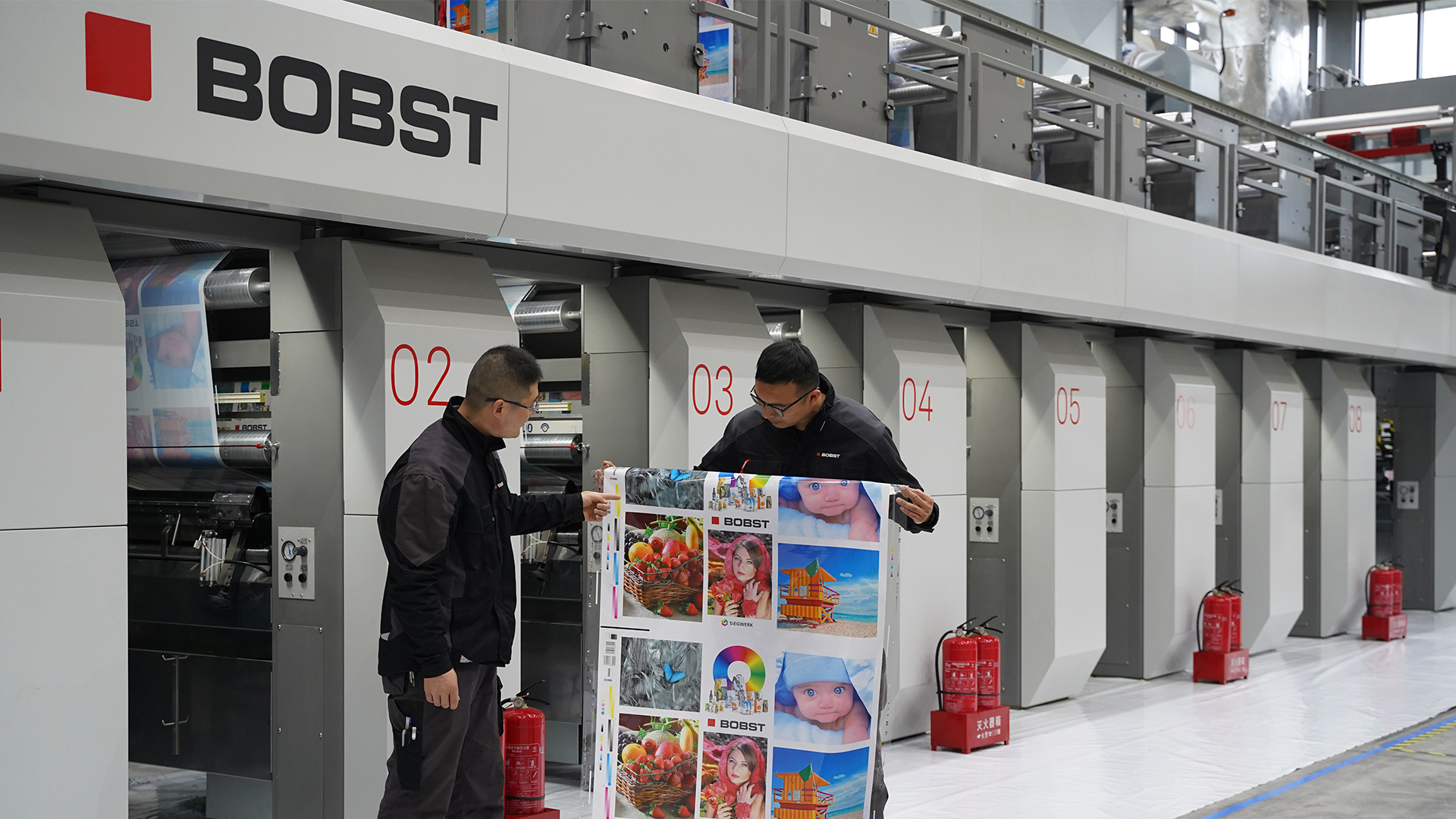In this detailed photograph, set inside an industrial print shop, two men are in the foreground, both wearing matching black jackets and glasses. They are inspecting a large colorful poster laden with various vivid images, including a baby in a blue cap, a red and green floral arrangement, a blue butterfly, a beach scene, a woman in a red headscarf, and a basket of fruit. One man points at the butterfly, while the other holds the poster.

The background features multiple printing machines housed in small open cubicles or rooms. Red fire extinguishers accompany each pillar, which are sequentially labeled as 02, 03, 04, 05, 06, 07, and 08. Overhead, a walkway with grey metal railings can be seen, as well as overhead scaffolding. Prominently displayed on the back wall in bold black print is the word "B-O-B-S-T," accompanied by a red square. This likely indicates the brand or name associated with the printing facility.